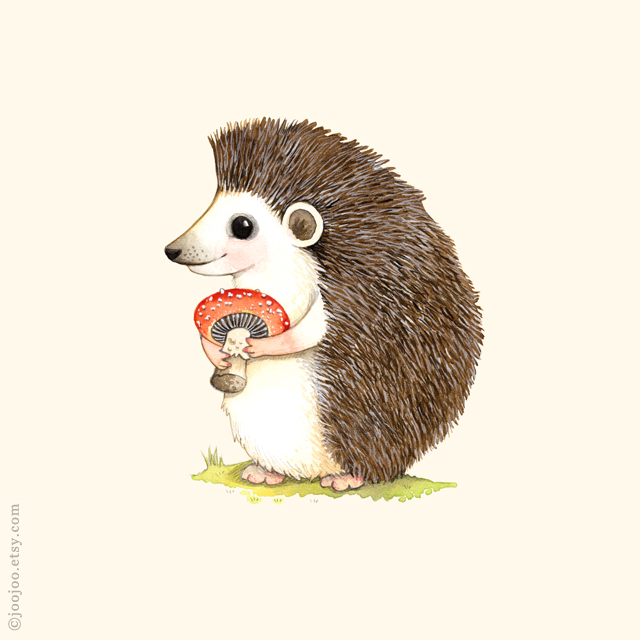A whimsical drawing depicts an anthropomorphized hedgehog standing upright on a small patch of green grass. The background is off-white, accentuating the central character's details. The hedgehog features a vibrant white face with a large black eye, framed by a touch of pink around the eye and brown near the small black nose. The inside of its ear is also brown. Its body transitions into a white belly and arms, with the same white hue extending to its feet, which have visible pink toes. The spines on its back are a mix of brown, white, and yellow, giving it a dynamic, wiry look. This charming creature is holding a striking red mushroom with white spots, distinguished by a dark gray stalk and a white stem. The hedgehog’s friendly expression, characterized by its smile and expressive eyes, adds to the overall endearing quality of this detailed and colorful illustration.